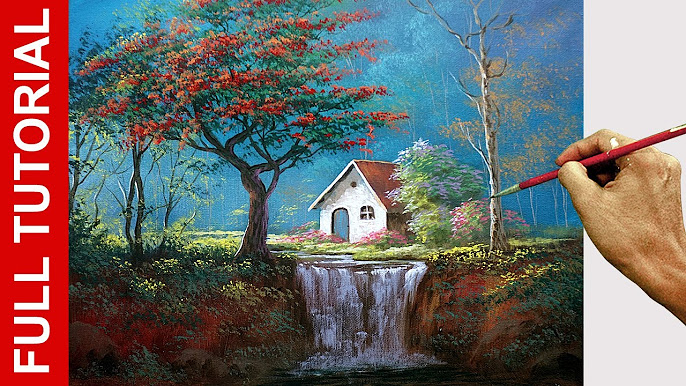The image appears to be an advertisement for a painting tutorial, showcasing a picturesque, detailed scene. On the left side, a vertical red stripe displays the text "full tutorial" in white lettering. Centrally, a hand entering from the right holds a red paintbrush, actively adding details to a painting on a white canvas. The scene being painted is of a quaint, white cottage with a red roof and blue door, featuring a window with a cross pattern. The cottage is surrounded by lush, colorful nature, including several trees. 

One tree to the right of the house is bare, while another to the left boasts red and green foliage, indicating autumn. Vibrant flowers, both purple and pink, bloom around the house, which is positioned above a flowing stream. This stream cascades into a waterfall in the foreground. The painting style is impressionistic, reminiscent of Thomas Kinkade's work, creating a whimsical, cottage-core, and fairy-like aesthetic. The sky is a vibrant blue with few clouds, enhancing the enchanting atmosphere of the scene.